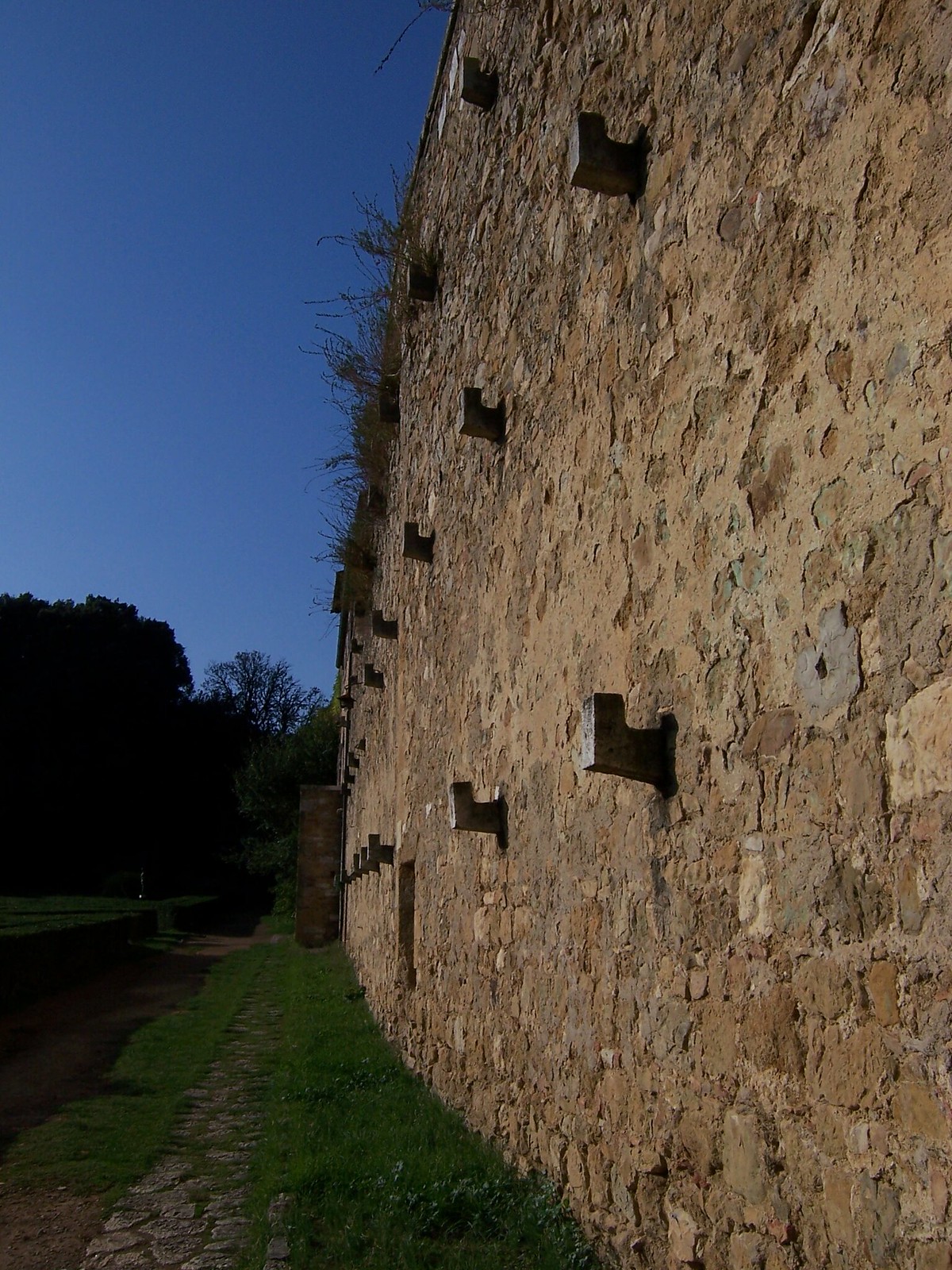In this outdoor image taken on a bright, clear day with blue skies, a tall stone wall dominates the right side of the frame. The light brown cobblestone wall, approximately three stories high, appears aged and weathered, with chipping and overhanging brush at the top. Metal hooks, possibly used for climbing or some historical purpose, are evenly spaced along its length. The wall stretches into the background, where a small entrance is barely visible. In front of the wall, a cobblestone walkway, slightly overgrown with grass, meanders towards the structure. On the left side, a lush green hedge garden leads to tall trees in the distance. Despite the bright setting, a dark area, possibly the shadow of a moat, is present on the left-hand side.